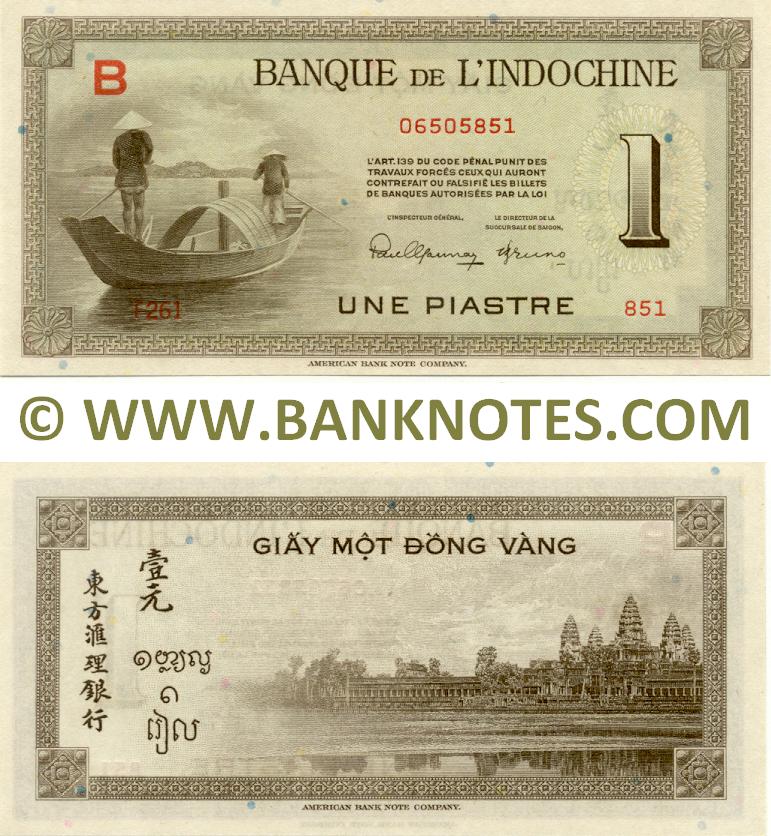The image displays a detailed view of the front and back sides of a $1 banknote from Indochina. The top half of the image showcases the front side of the note, labelled "Banque de l'Indochine" with the serial number 06505851, accompanied by a law article and a signature. Prominently featured on the left side is an illustration of two figures in a small boat, donning traditional East Asian conical hats, and navigating with long sticks across a river. The number "1" appears on the right side of this front view. The color scheme of the banknote includes light brownish-gray tones with green text indicating the source as www.banknotes.com. Below, the back side of the note is displayed, which exhibits a grand temple-like structure reminiscent of Angkor Wat, complete with ornate towers and spiked details. Surrounding the image of the building, there is text in various languages, including Chinese, Vietnamese, Thai, and possibly Lao, with the note being manufactured by the American Banknote Company.